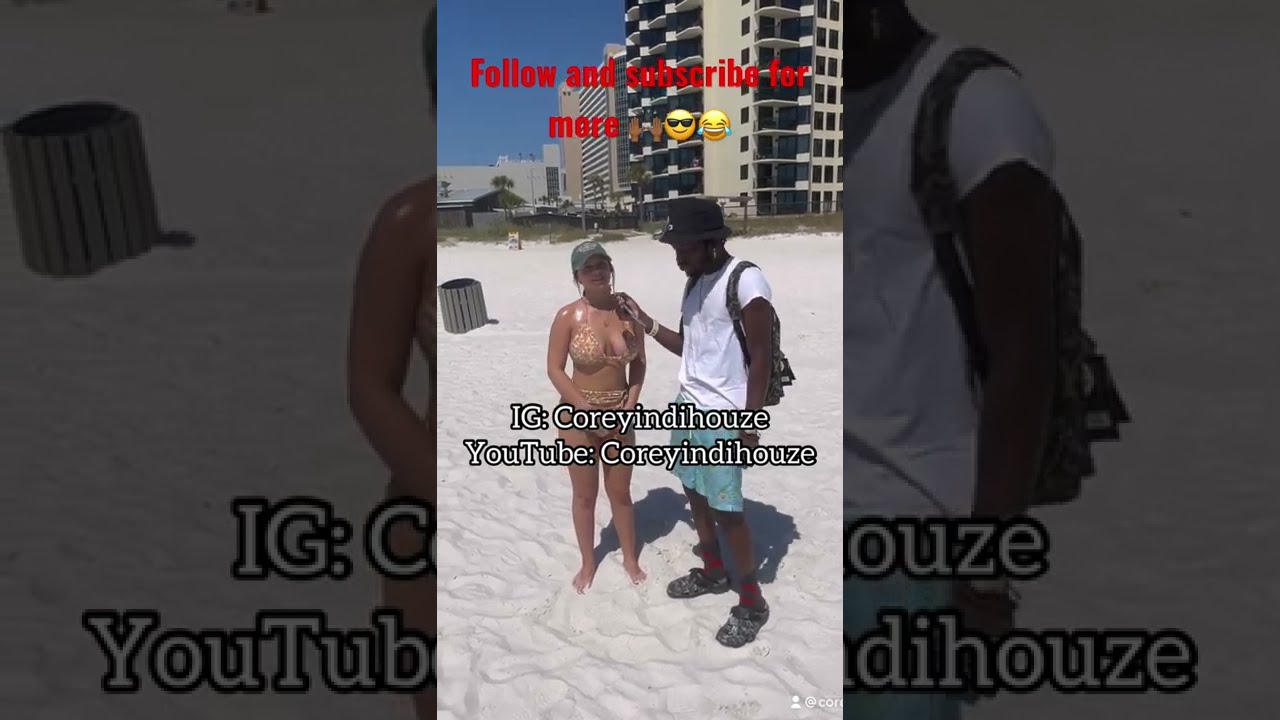The image depicts a man conducting an interview with a woman on a sunny beach, with beach condos visible in the background. The man, an African-American, is dressed in a white t-shirt, green shorts or teal pants, black Crocs or sandals, red socks, and a black bucket hat. He also sports a black backpack and a bracelet. He is holding a microphone up to the woman, who is standing to his left. The woman is wearing a gold and white bikini and a green or gray baseball cap, with her head turned to the right as she responds to his question.

There is white text over the image that reads "IG: Corey Indy who's? YouTube: Corey Indy who's," along with the top text in red font saying, "follow and subscribe for more." The text is accompanied by emojis, including hands high-fiving, a smiley face with sunglasses, and a laughing-crying face. The context implies it might be a clip from an internet video or social media content where random people are interviewed or participate in challenges. Additionally, a garbage can is visible in the sand, enhancing the beach setting.